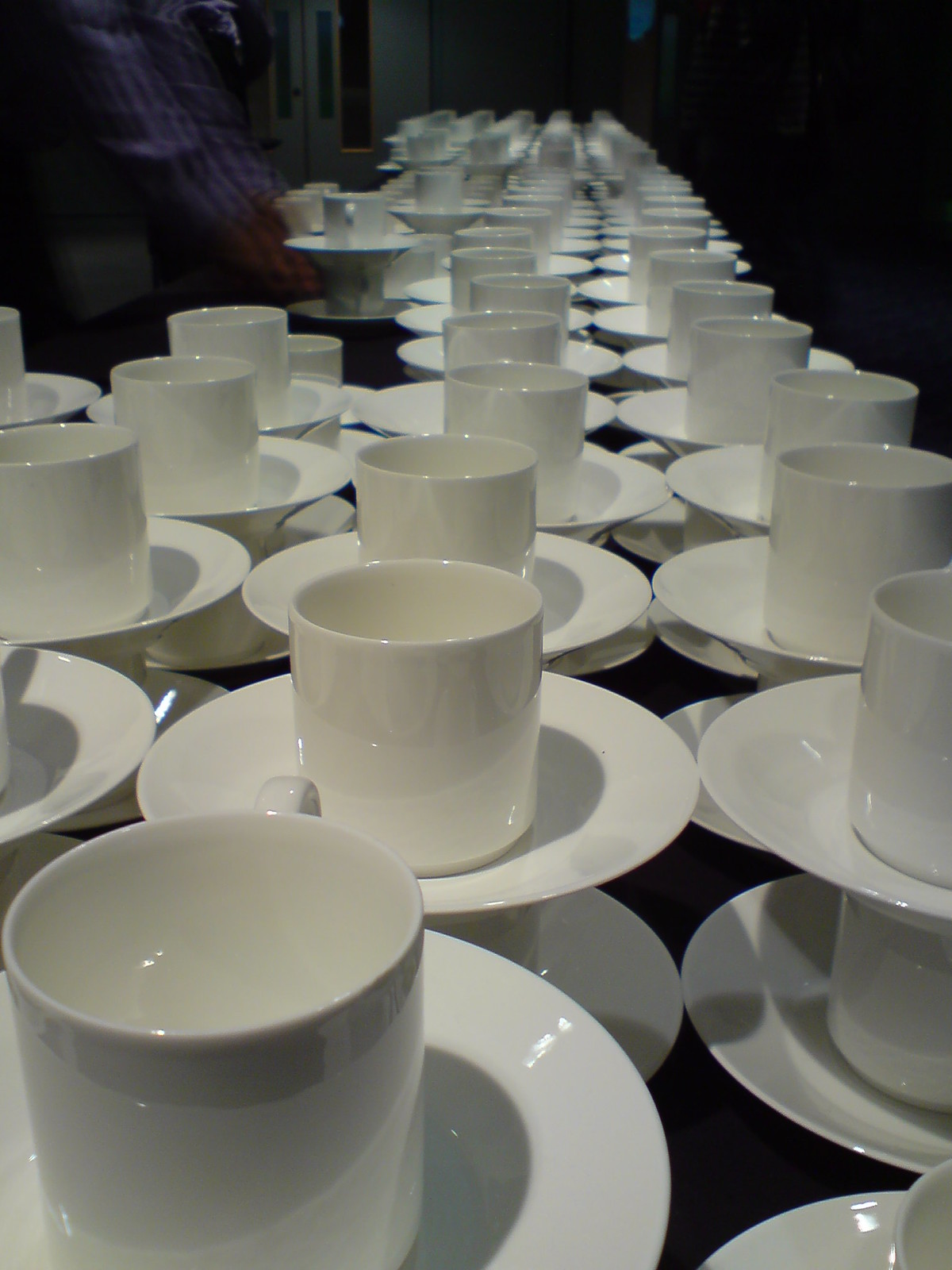The photograph is a realistic, vertical rectangular shot taken indoors with dark, ambient lighting. The main focus is a long black table covered meticulously with high stacks of white ceramic tableware. Each stack comprises a white saucer, topped by a white mug, followed by another saucer and mug, creating a series of double-stacked cups and saucers. These stacks, all identical and glossy, extend horizontally in rows of four and retreat back further than the eye can see, amounting to at least 20 or 30 rows. The blurred background reveals a white door on the back left and hints at human presence; a blurry arm is seen reaching from the left, clothed in a blue checkered shirt, perhaps unsettling one of the stacks. Despite the table's orderly arrangement, the dark surroundings and the motion blur add a dynamic, somewhat mysterious feel to the scene.